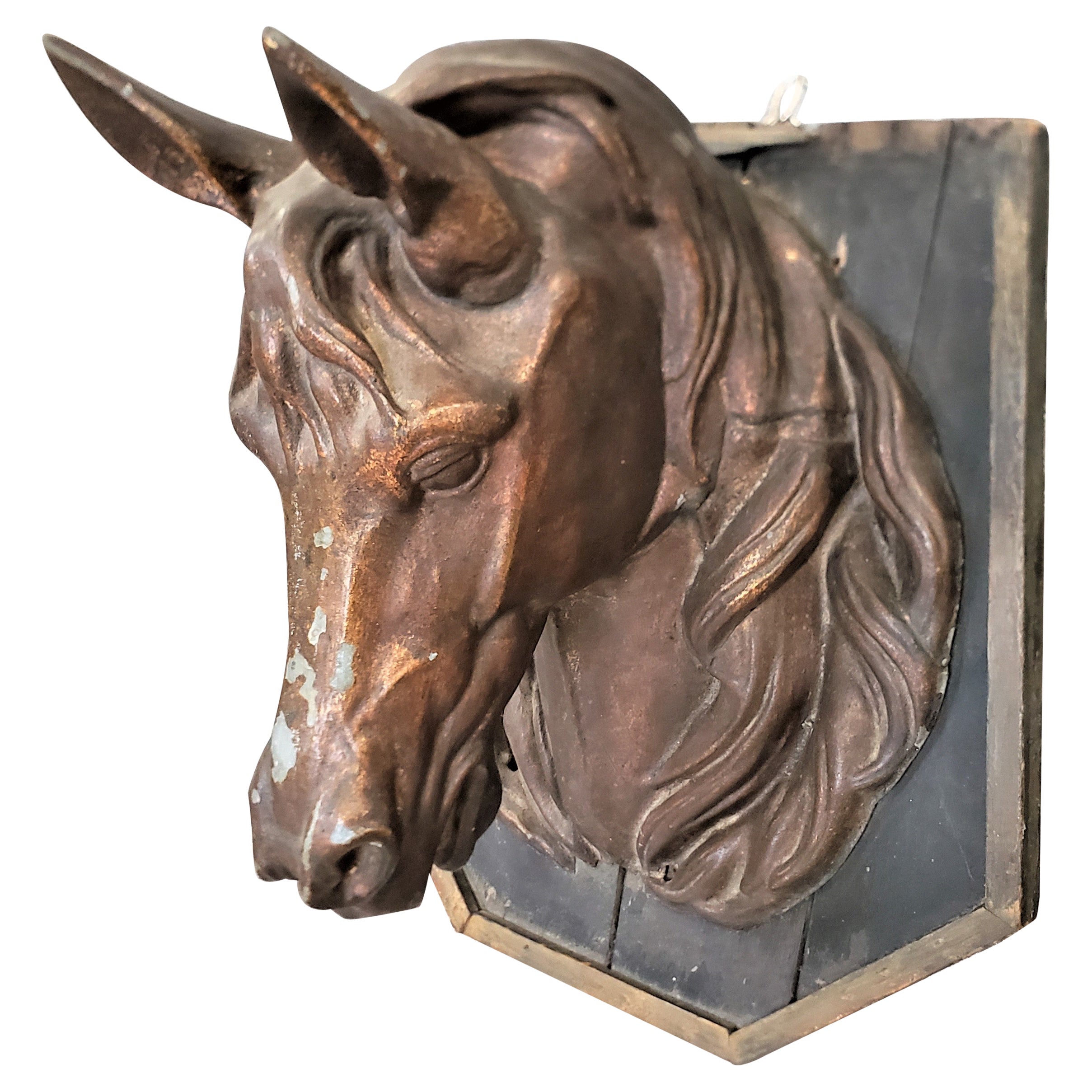The photograph showcases an aged horse head sculpture, made from what appears to be bronze or a similar metallic material, affixed to a wall. The sculpture captures the head and mane of the horse, with its ears protruding outward and its eye closed, giving the impression of a serene, downward gaze as if the horse is sleeping. The head is turned to the left, with some rust present near the eye and visible peeling on the nose, suggesting its antiquity. The sculpture is mounted on a dark wood plaque, bordered in a lighter brown wood, enhancing its classic appearance. A small hook is visible at the top of the plaque, designed for hanging. The backdrop is a white wall, accentuating the darker hues of the sculpture and its wooden frame.